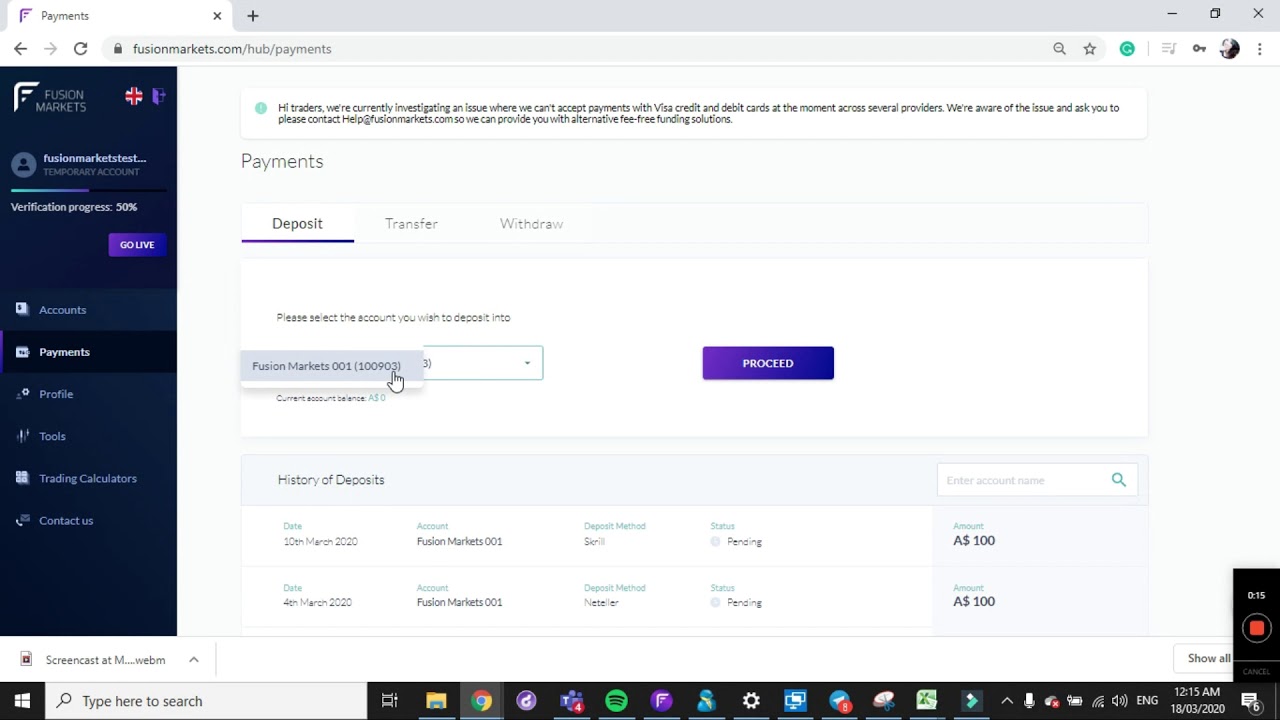This image depicts a webpage from Fusion Markets. In the top left corner, the active tab labeled "Payments" is visible. On the top right, there are three navigation buttons: minimize, full-screen, and close (X). Below the "Payments" tab on the left side, there are three more buttons: back, forward, and refresh. Directly to the right of these buttons is a search bar featuring a lock icon on the left, followed by the URL "FusionMarkets.com/hub/payments."

Immediately beneath the search bar, there is a block of text addressing traders: "Hi traders, we're currently investigating an issue where we cannot accept payments with Visa credit and debit cards at the moment across several providers. We're aware of the issue and ask you to please contact help@FusionMarkets.com so we can provide you with alternative fee-free funding solutions."

Further down, the section is labeled "Payments," under which there are three available options for the users to select.